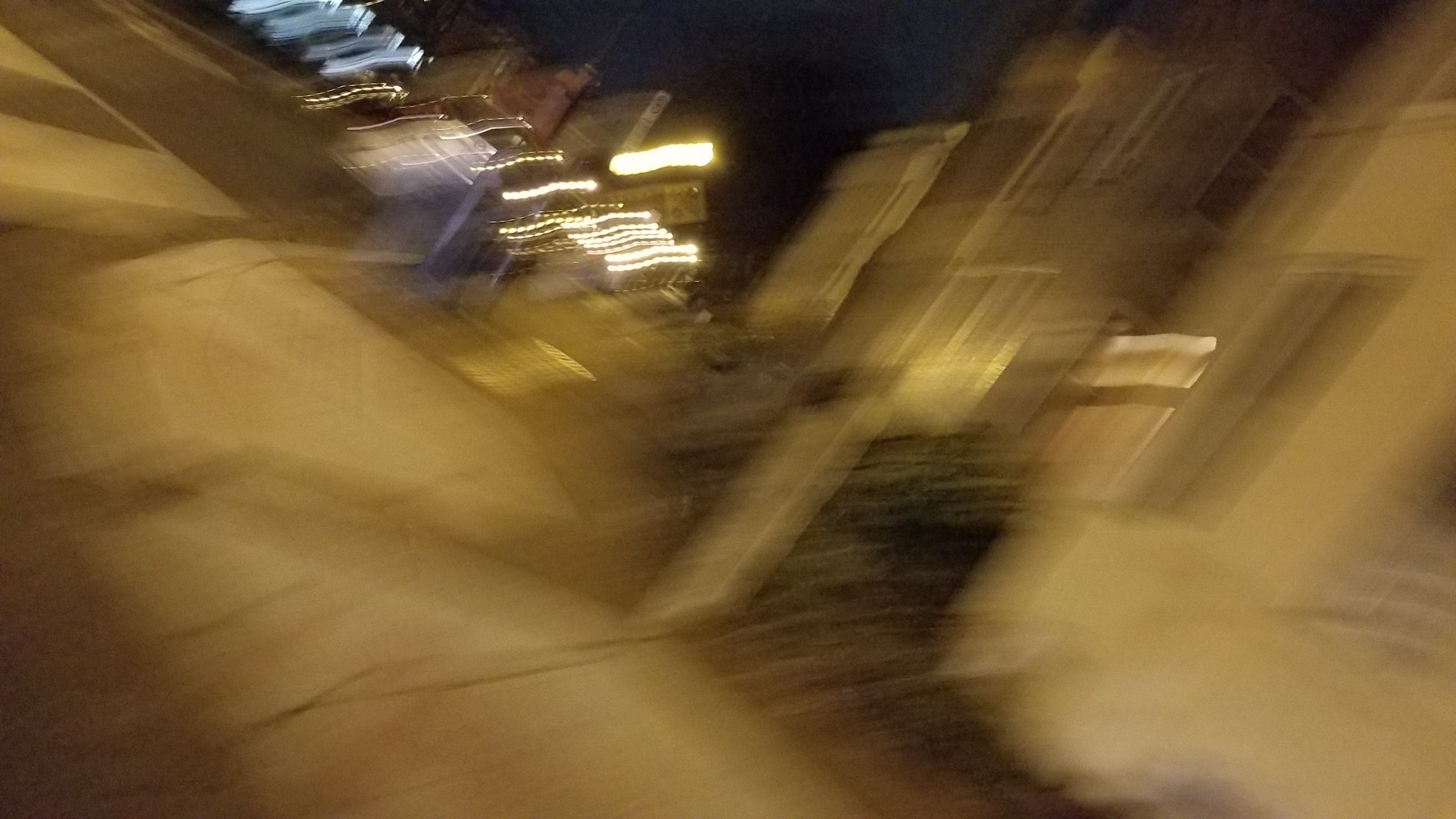In this image, a distinctly out-of-focus and blurry scene makes it challenging to discern specific details. However, it appears to capture an urban vista with several buildings that appear to be a brownish-gray hue. On the right side of the image, there is a faint outline of a sidewalk, colored in a nearly gray shade which matches the hazy tones of the buildings nearby. Dominating the upper portion of the photo, various streaks of light in different colors streak across the scene. These include prominent white light streaks, accompanied by blurry blue lights both to the left and interspersed among the white lights. Further up, beyond these streaks, the faint presence of the night sky is suggested, adding to the overall sense of disorientation and mystique in this photograph.